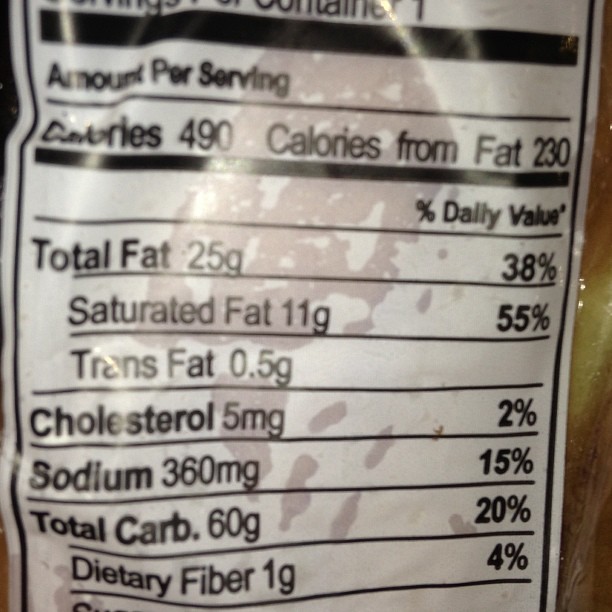This image is a close-up of a black and white nutritional facts label attached to a possibly transparent, slightly crumpled, and moisture-splotched packaging, revealing glimpses of a light brown product inside. The top part of the label is cut off, but you can make out "servings per container: one" and "amount per serving." Below this, the clear text indicates 490 calories per serving, with 230 calories from fat. Nutritional details include 25 grams of total fat (38% daily value), 11 grams of saturated fat (55% daily value), and 0.5 grams of trans fat. The label also lists 5 milligrams of cholesterol (2% daily value), 260 milligrams of sodium (15% daily value), 60 grams of total carbohydrates (20% daily value), and 1 gram of dietary fiber (4% daily value). The label is sectioned by thick and thin black dividers, with items listed in a mix of bold and regular black text. The edges show the cellophane wrapper, with the label sticking to the packaging, adding splotchy grayish areas.